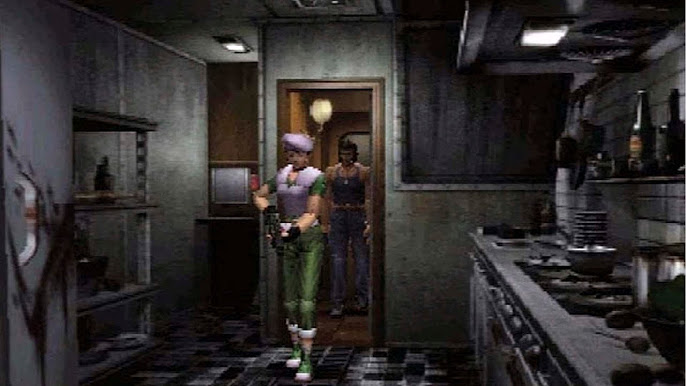This detailed image is a screenshot from the video game Resident Evil 3, featuring the characters Jill Valentine and Carlos Oliveira. The scene takes place in a barren and bloody kitchen with silver, metal-like walls and a muted shelving unit on the left, consisting of four shelves. On the right side, there's a stove and another shelf, with the floor exhibiting a black and gray pattern. An overhead light shines down on the stove area.

Jill Valentine is distinctly dressed in a non-traditional outfit, wearing green pants, green high-top tennis shoes, a purple vest, and a purple hat, deviating from her usual blue attire. She's holding a gun in her hands, adding to the action-oriented theme of the game. Accompanying her is Carlos Oliveira, who has shoulder-length black curly hair and a muscular build, adorned in a grey tank top with a dog tag necklace and blue jeans. 

Amidst the kitchen decor, there are visible oven dials, a stack of plates, a couple of bottles on the right shelf, and fans and lights at the top right. The two characters are seen entering through a central doorway, emphasizing their exploration of this metallic, desolate room indicative of the survival horror atmosphere of the Resident Evil series.